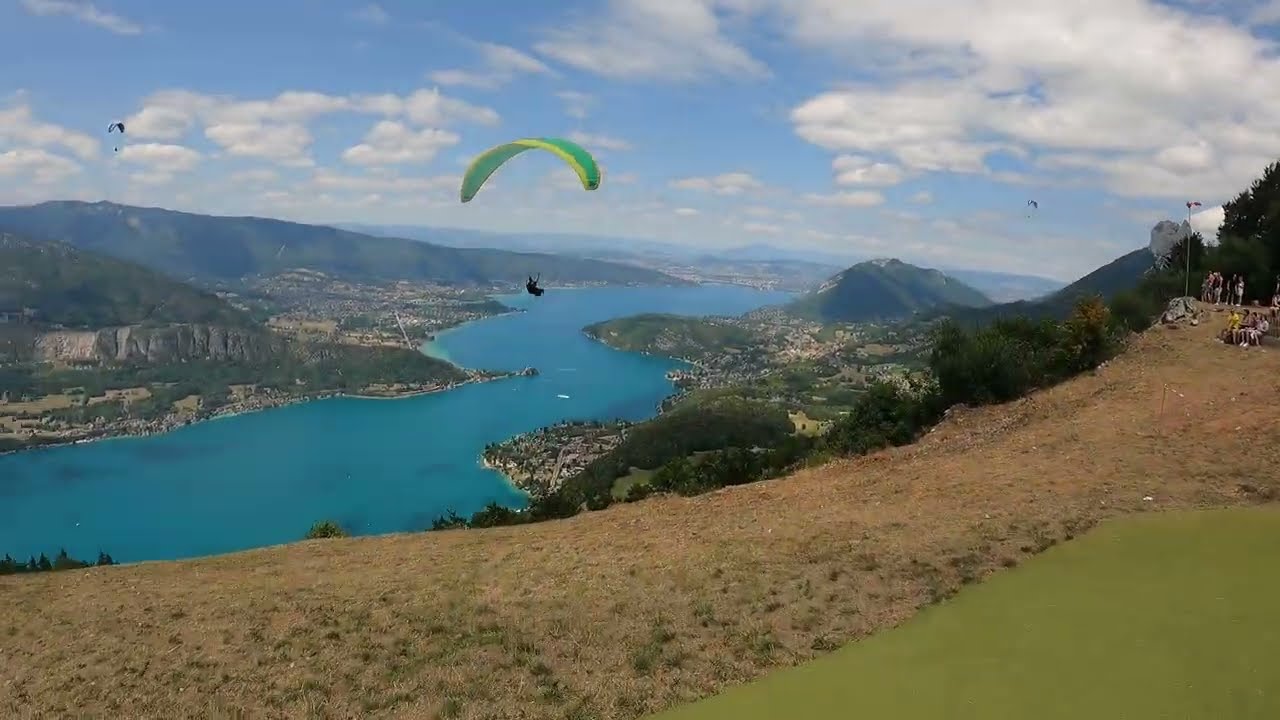The image showcases a picturesque, elevated view of a lush valley surrounded by majestic mountains and hilltops. A glider is seen gracefully descending towards the vibrant landscape, which is dotted with verdant green fields and small, distant towns. These towns are nestled beside a meandering river that snakes through the valley, forming a captivating reverse C shape where it is punctuated by two distinct points of land. The largest town lies further in the distance, framed seamlessly by the mountain range.

In the foreground, a green mat is visible on the mountaintop, providing a stable platform amidst the grassy terrain. The scene is lively with several people either standing or sitting, possibly hikers or fellow gliding enthusiasts, observing the glider’s descent. Additionally, two parachutists are captured in the shot; one with a green parachute is closer to the viewer, while another with a white parachute is further off, creating an interesting dynamic in the sky.

The sky above is dotted with clouds, adding a dramatic backdrop to the serene yet bustling valley below. The image powerfully conveys the thrill of adventure and the serene beauty of nature, capturing a moment of harmonious interaction between humans and the expansive landscape.